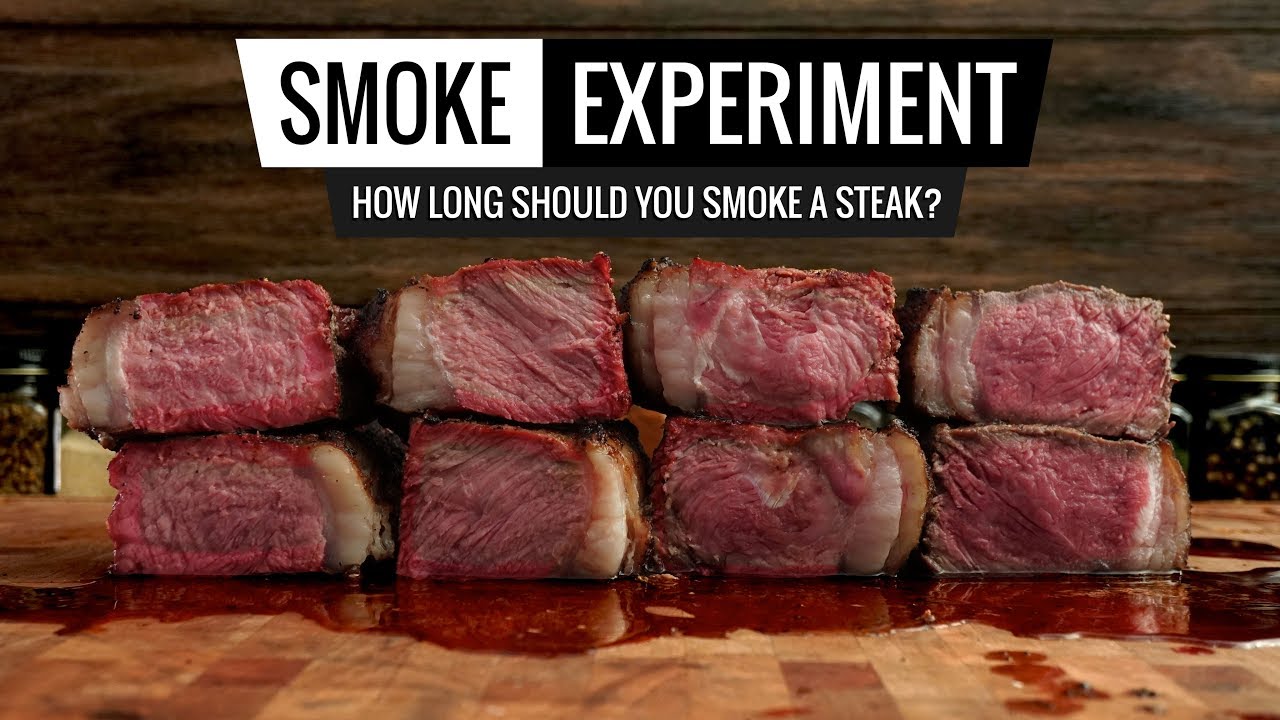The image is a horizontally-oriented photograph prominently featuring eight cuts of steak, stacked in two rows of four on a wooden butcher board. The steaks, sliced to reveal their medium-rare to medium-well interiors, show intricate marbling and fatty sections, with juices visibly pooling around them, suggesting fresh cuts. The background consists of dark, weathered wood paneling, with a hint of spice bottles visible on the left side, slightly out of focus. Dominating the top portion of the image, black and white text reads: "Smoke Experiment: How Long Should You Smoke a Steak?" with alternating color schemes where necessary.